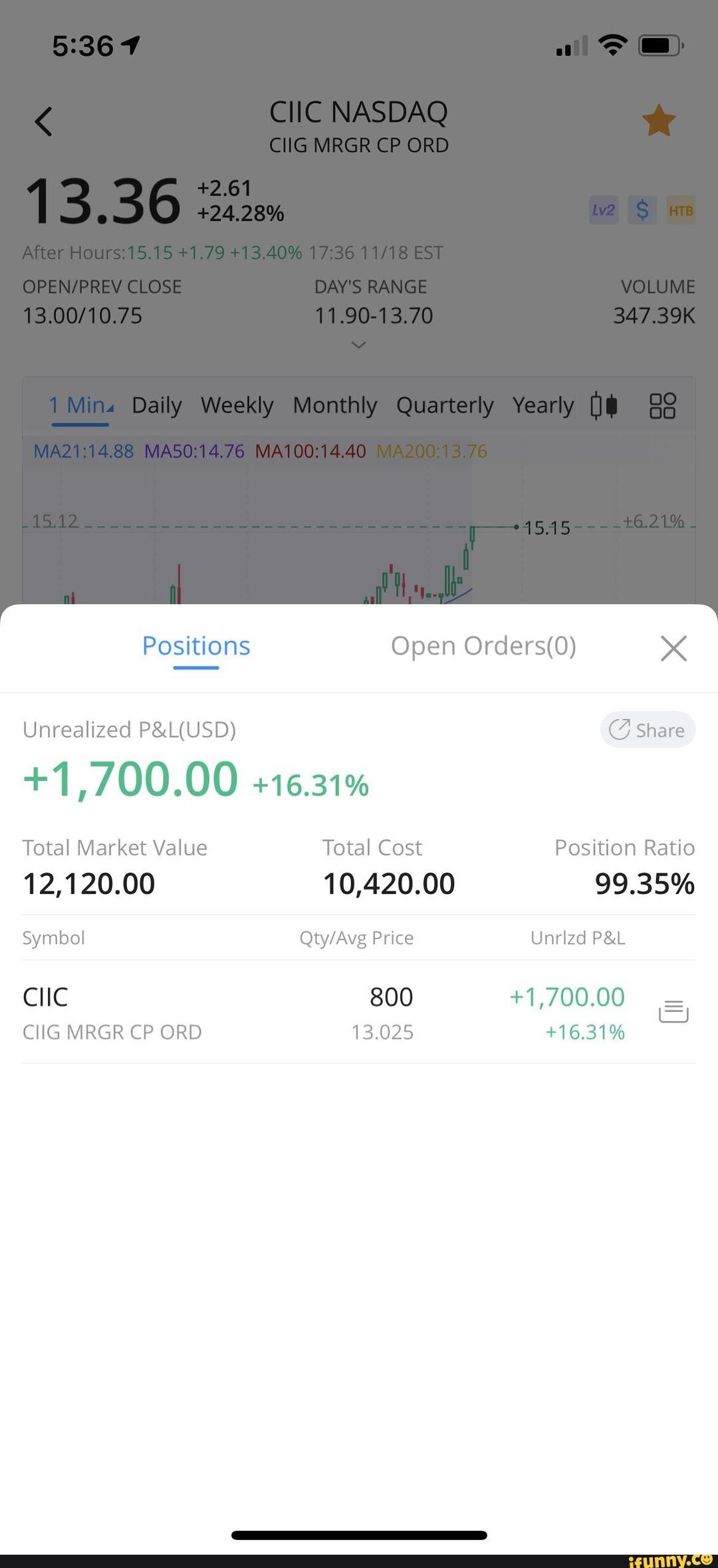This caption needs to be refined and detailed. Here's a polished version:

---

This image appears to be a screenshot from a mobile trading app. The screenshot has a grayed-out background with an overlay of a white rectangle, indicating that a menu or detailed view is being pulled up. The top half of the image is a static screen displaying various financial statistics. 

In the top section, there is a series of black texts with the heading "Click NASDAQ CHG MRGR CP or D" followed by different numerical values. Below it, a bold figure '13.36' stands out prominently against the rest of the text. Underneath, there are labels such as "Open," "Previously Close" with respective numbers '13.00' and '10.75'. The section also displays "Day's Range" alongside other key metrics such as trading volume.

A partial line graph is visible, labeled with different time periods: Daily, Weekly, Monthly, Quarterly, and Yearly, although only the very top of the graph is seen. 

The overlying white rectangle reveals an active menu with tabs "Positions" and "Open Orders," where "Positions" is selected and highlighted in blue. This section contains financial data, stating "Unrealized P&L USD" with a gain of '1700.00' and '16.31%,' also in blue. Additional information includes "Total Market Value" of '12,120,' "Total Cost" of '10,420,' and "Position Ratio" of '99.35%.' 

Further, the app lists a stock or entity named "CICC" with unclear accompanying text. Positioned in the middle of this tab is the number '800,' and another gain of '1700.00' and '16.31%,' albeit in smaller blue font.

Space beneath this data remains blank, highlighting the contrast between the detailed metrics and the white background of the interface.

---

This revised caption captures all key details and arranges them coherently.